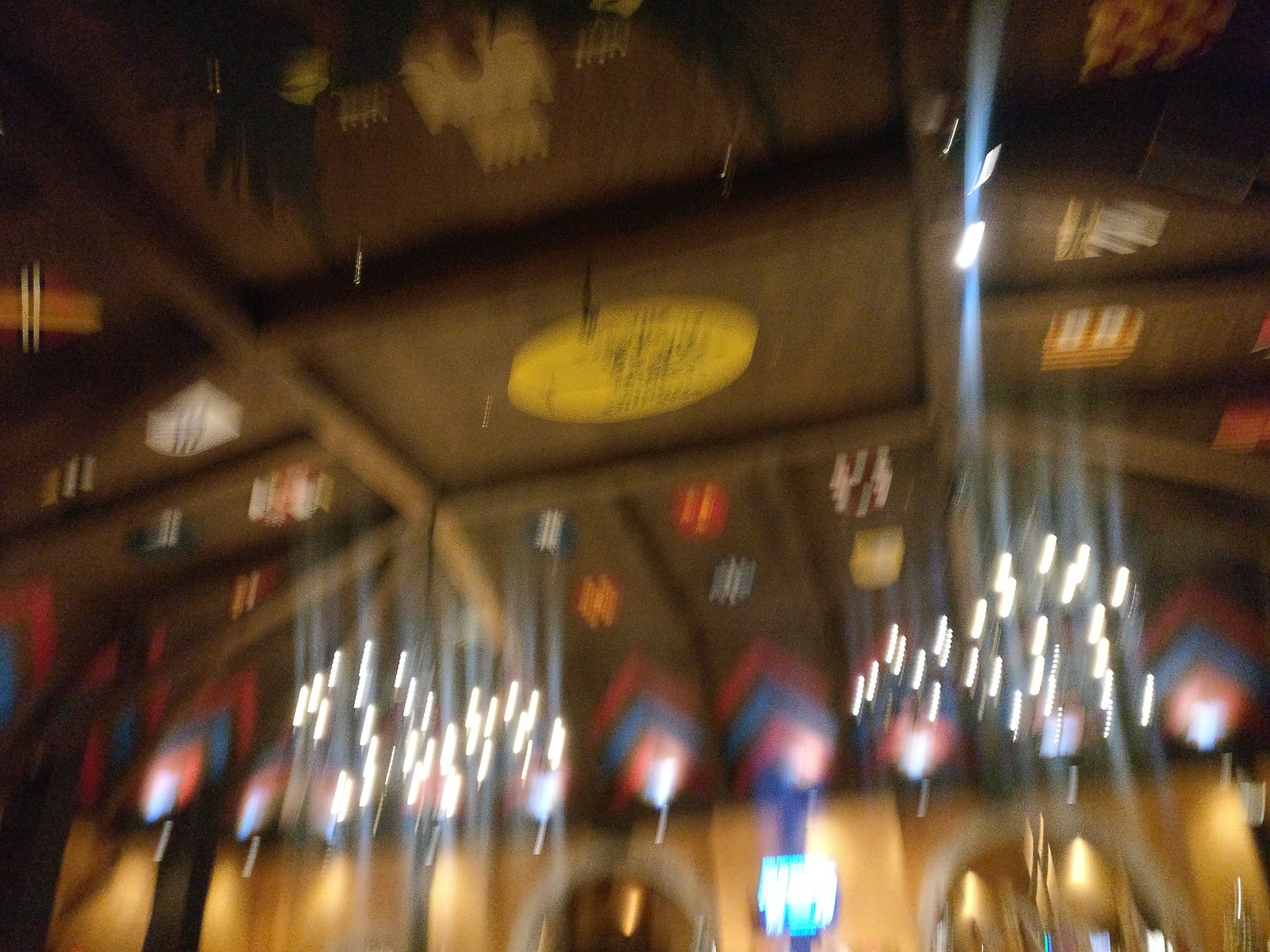This highly blurred photograph features an array of indistinguishable black shapes, some resembling rectangles while others take on more square forms. The lighting appears distorted as if the camera was in motion during the capture, resulting in streaks of light. These light streaks, resembling small dashes, are concentrated in two distinct clusters in the bottom third of the image. Additional lights are dispersed sporadically around the edges. At the center of the upper section of the image, there is a square shape with a yellow circular detail within it. Along the bottom, the rectangular forms are marked with red and blue chevron patterns. The entire scene is primarily dominated by black shapes intermixed with sporadic, colorful details, all shrouded in a sense of mystery due to the image’s lack of clarity.